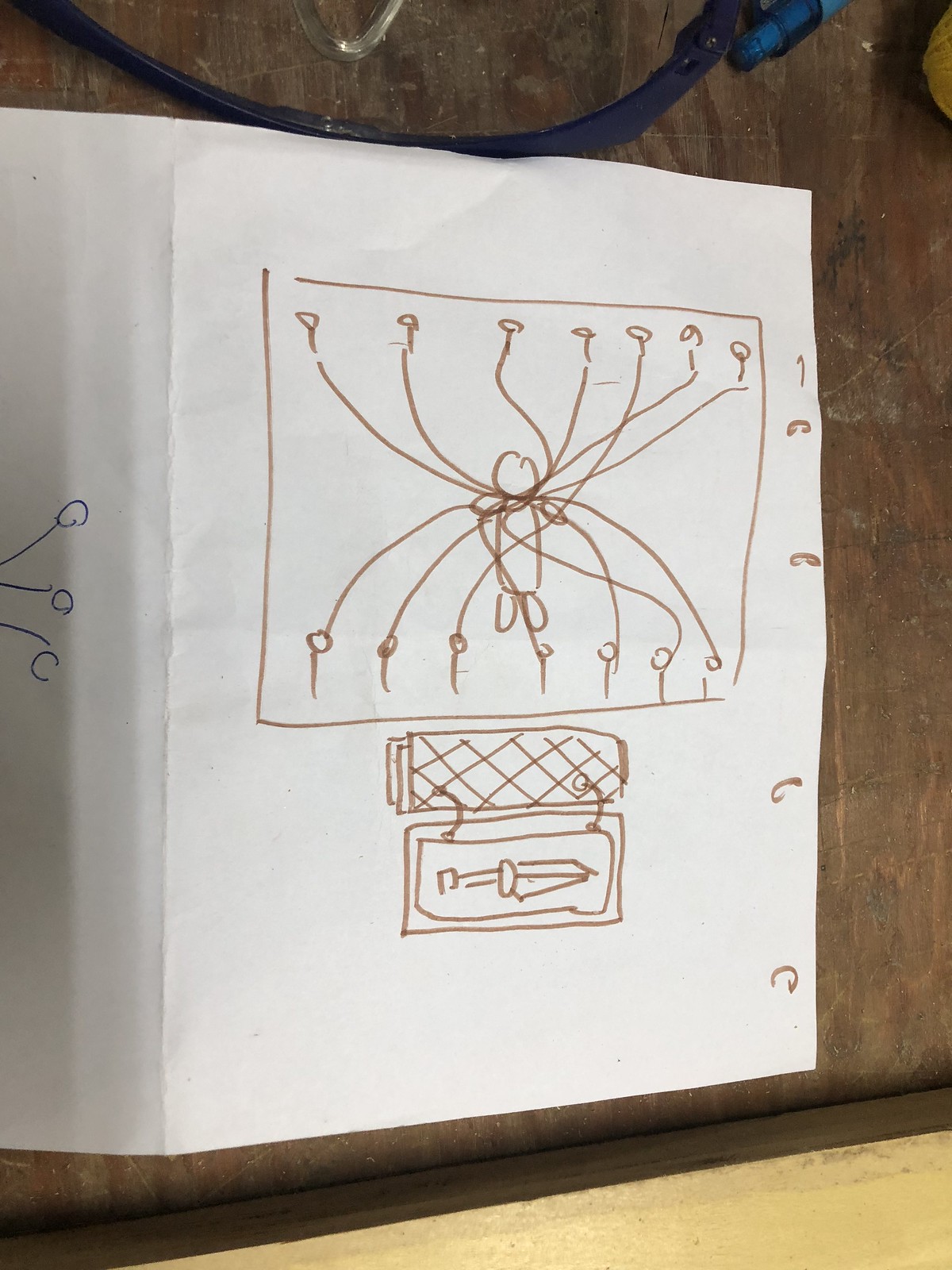This photograph captures a detailed drawing executed by a competent artist, suggesting significant experience beyond that of a novice or child. Rendered on notebook paper, the image partially reveals another drawing on the left, with three arm-like structures extending from the right, each ending in circular forms.

The focus of the photograph is the main drawing situated centrally. It depicts a figure, resembling but more complex than a traditional stick figure. The figure's limbs consist of circles, with the arms and legs fully formed by these circular shapes. The body is illustrated as an oval, and the head is a distinct circle.

Extending from this figure are multiple devices resembling wires, which connect both to the top and bottom of the figure. These wires terminate in circles at each end, suggesting points of connection or control. At the base of the drawing, there appears to be an open case or container, intricately designed with a cross-stitch pattern. Inside, a knife is prominently displayed, resting within the case. The arrangement of the elements and the meticulous detail suggest a narrative or conceptual depth within the artwork.